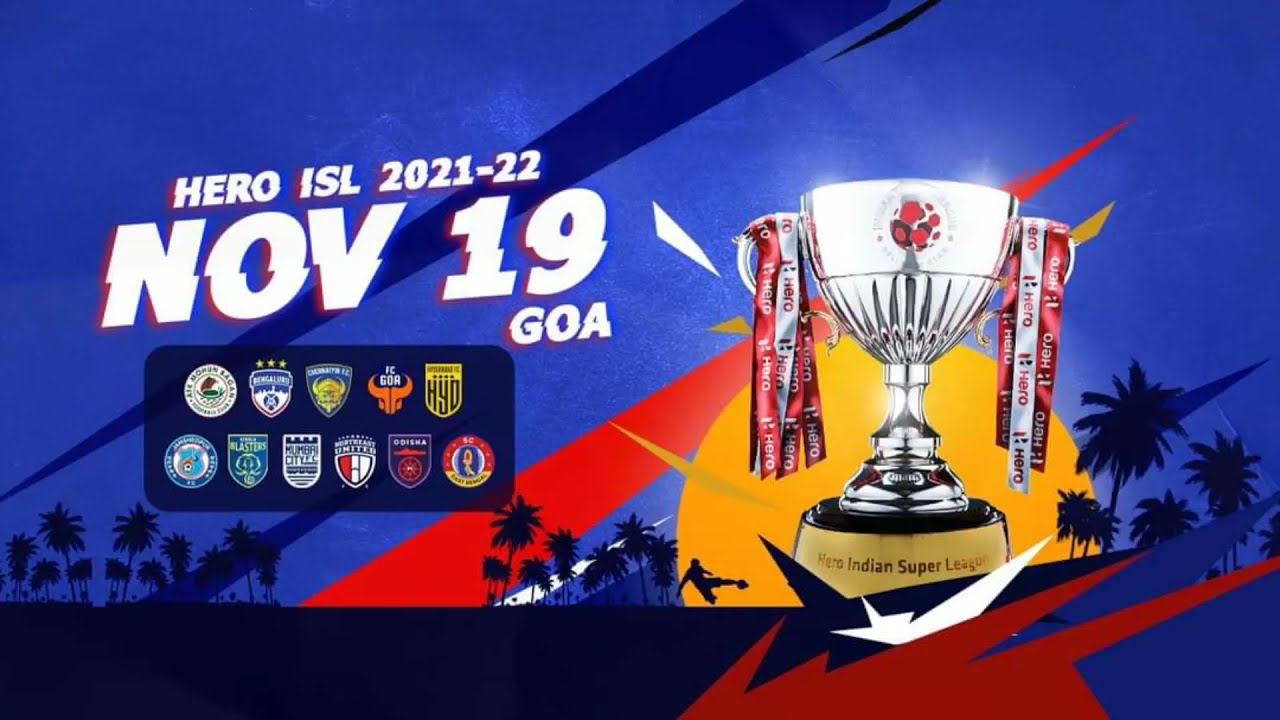The image appears to be an advertisement for the Hero Indian Super League 2021-22, scheduled for November 19th in Goa. It is horizontally rectangular with a rich blue background that transitions into a darker blue toward the top, simulating a night sky. Diagonal stripes in dark blue and red emerge from just right of center, adding dynamism to the composition. At the bottom of the image, a row of palm trees is silhouetted in dark blue. Centrally located text in white reads "Hero ISL 2021-22 NOV 19 GOA" at an angle, left to right. Adjacent to the text, to the right, is a prominent silver trophy adorned with red and silver ribbons. The trophy is positioned against an orange-yellow setting sun, with the base featuring the words "Hero Indian Super League" in black lettering. In the lower left corner, a small black rectangle contains various circular and shield-like symbols, resembling patches. The overall design is vibrant and rich with elements emphasizing a tropical, celebratory atmosphere.